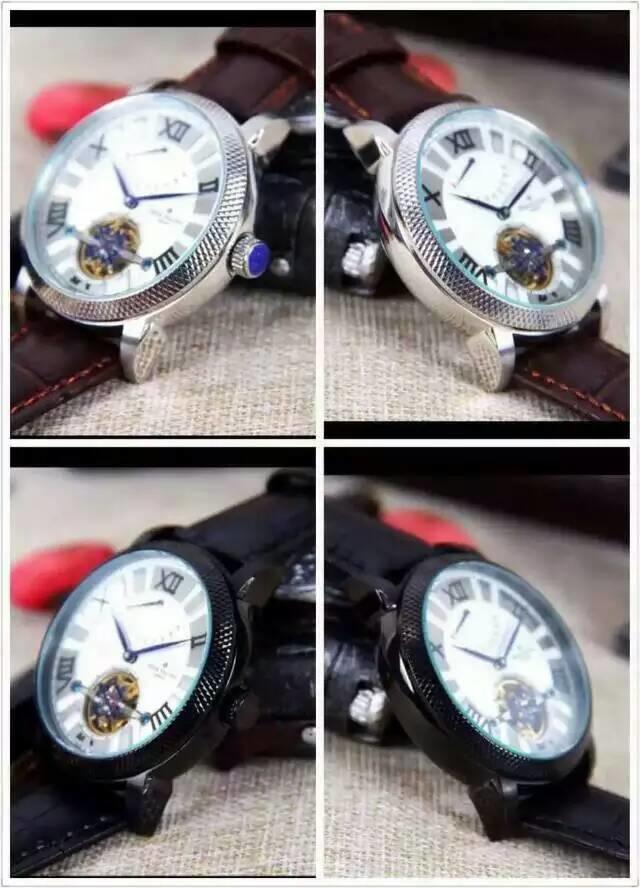A detailed description of the image:

The image showcases a grid of four square photographs, each depicting a watch face from different angles, all set against a gray, carpet-like surface. The background also contains a recurring blurred red circle. 

1. **Top Left Image**: This watch features a white face with a silver lining. On the side, there is a twist knob with a distinctive purple tip. The watch is complemented by a brown wristband.

2. **Top Right Image**: Displaying the same watch but from the opposite side, this photo highlights the golden circle in the center of its white face, along with subtle blue details. The twist knob is less visible from this angle.

3. **Bottom Left Image**: Similar to the watches in the top row, this watch has a black wristband and a black lining around the watch face. The design inside the watch face mirrors the golden and blue accents seen in the previous watch.

4. **Bottom Right Image**: This image presents the same watch as the bottom left, viewed from the opposite side. The black wristband and black lining are clearly visible, along with the golden circle and blue details at the center.

All watches share the same background elements and are likely variations of the same model, distinguished by their wristbands and lining colors.